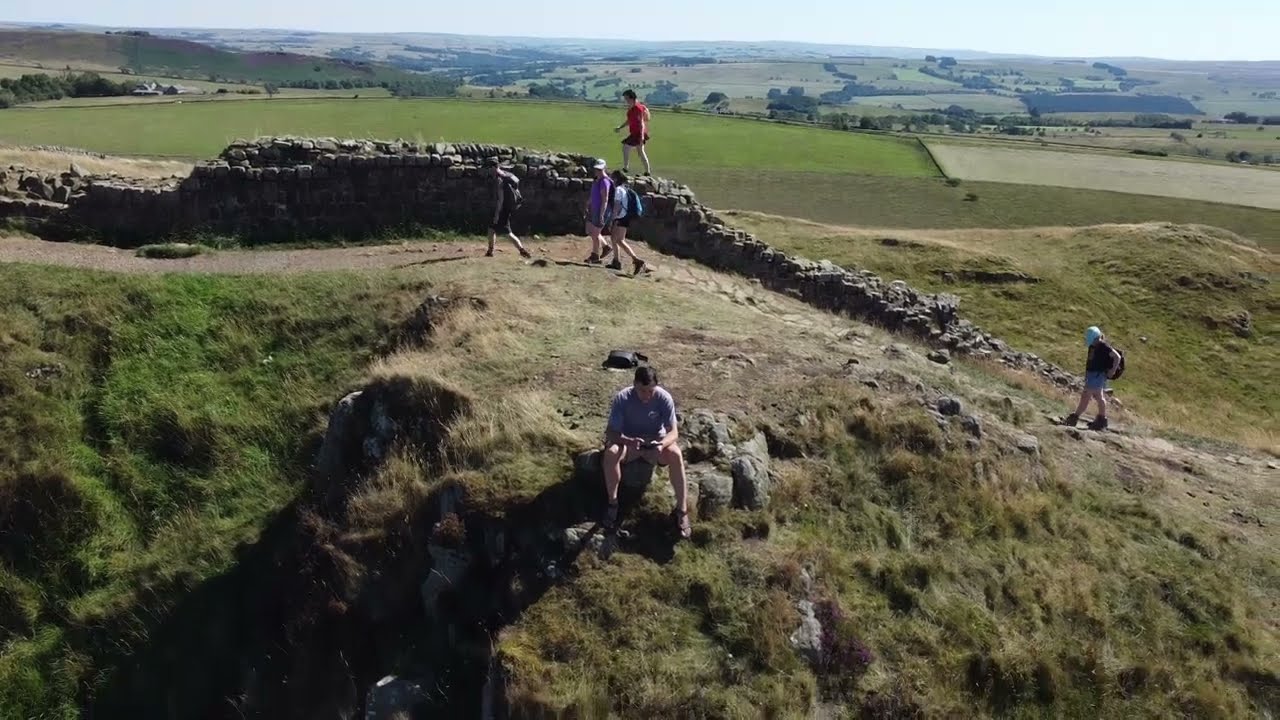The image depicts a group of hikers traversing a hilly landscape under a hazy blue sky. In the foreground, a stone wall, appearing old and crumbling, stretches horizontally. Alongside this wall, a dirt path extends from the right, ascends a small incline, levels out, and continues leftwards. On this path, near the crest of the hill, three hikers wearing backpacks and hiking gear are visible. One of them is standing on a section of the wall. 

A man in a blue shirt and shorts is sitting on rocks at a small outcropping of the path, seemingly resting or looking at his phone. The surrounding terrain features patches of dry and green grass, with a scenic vista of fields and farmland in the background. The midday sun casts a warm glow over the landscape, highlighting the varied textures of the grassy hills and the distant valleys.